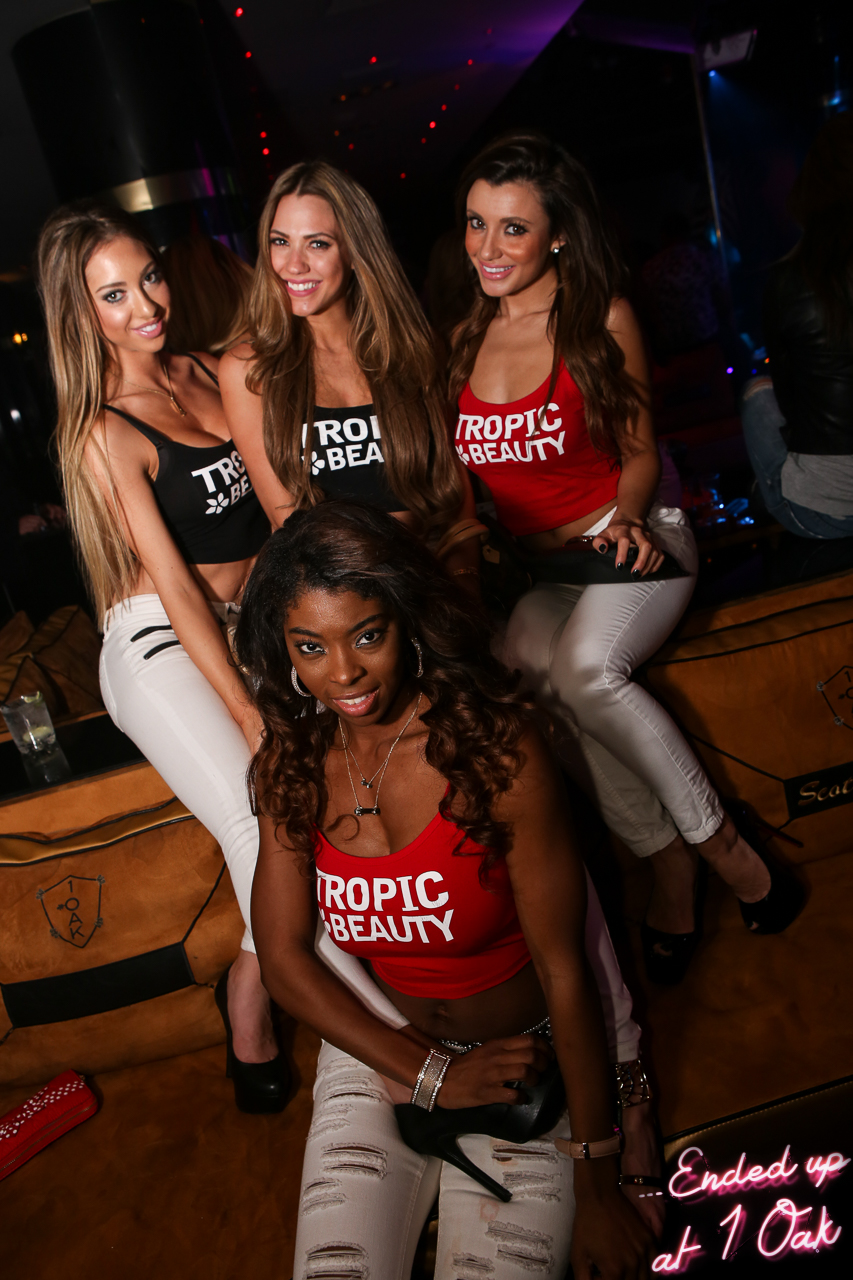This photograph captures a scene of four young women at nighttime, seemingly at a bar with an oak countertop or possibly an open rooftop setting. They are all sporting black and red tank tops with the words "Tropic Beauty" emblazoned on them in white text. Their attire also includes white ripped jeans and high black heels. Three of the women are sitting next to each other, positioned at the top of the image, while the fourth woman, who has darker hair, is seated at the bottom center of the image. The background is dark, accented with purple and red lights, evoking a nightlife atmosphere. A glass of alcohol can be seen to the left of one of the women. The bottom right corner of the photograph is marked with the text, "Ended Up at One Oak." The women all have long, lighter-colored hair, except for the woman with darker hair seated in the foreground.